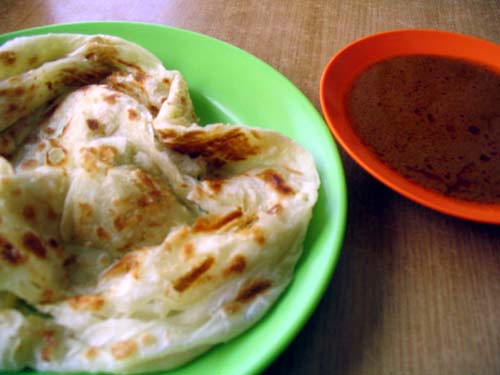This is a close-up photograph of food displayed on a wood grain tabletop with visible light highlights apparently coming from a window in the upper left-hand corner. On the left side of the image, a green plastic plate is partially cut off by the frame and holds a browned tortilla or a similar type of pastry, possibly containing cheese, although the interior is not clearly visible. The tortilla appears wrinkled and fully cooked. Adjacent to the plate, on the right, there is a shallow red plastic bowl containing a reddish soup or sauce, which might be tomato soup or chili. There are no people in the photograph, and the overall focus is purely on the food and the tabletop.